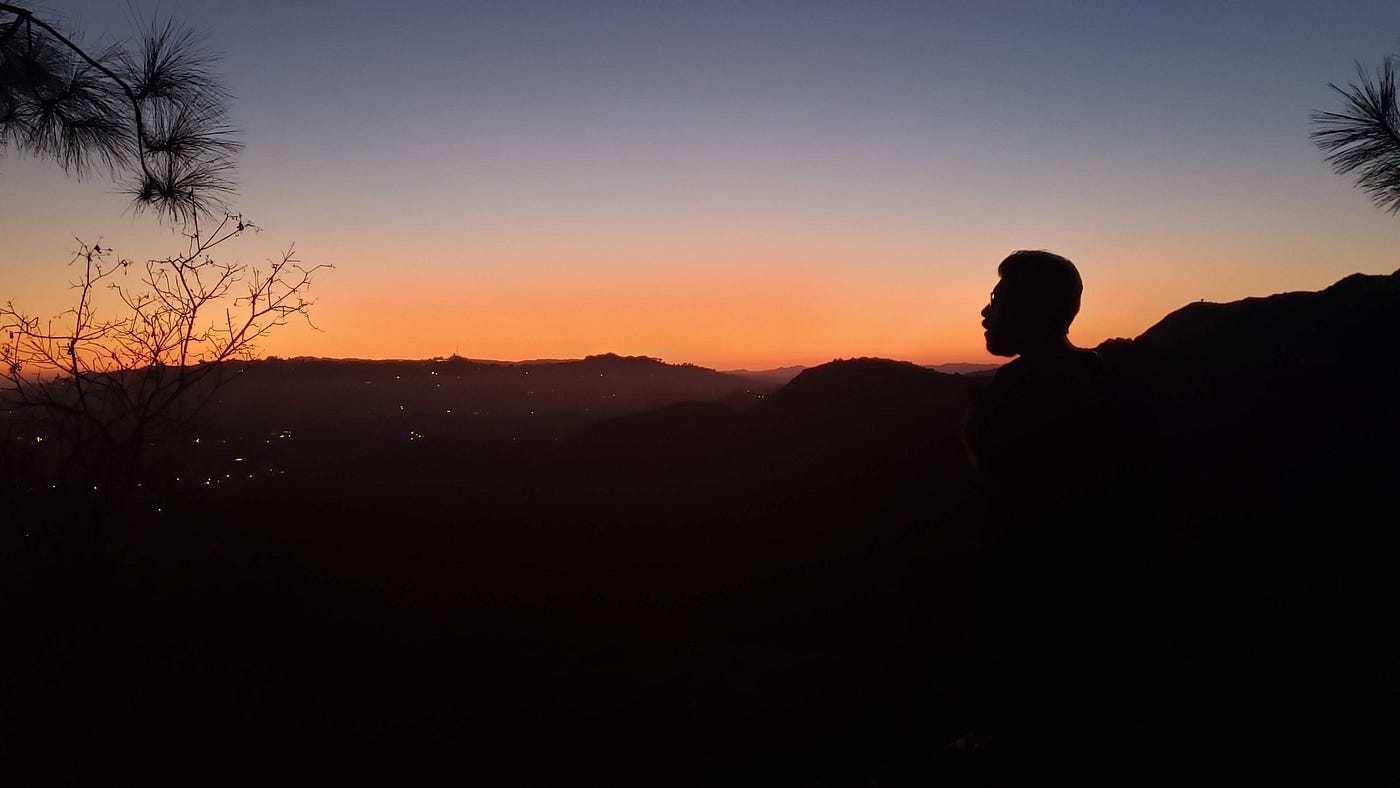The image captures a serene twilight scene transitioning from sunset to night. The sky at the top shifts from a deep iron blue down to a muted orange at the horizon, where the Sun is setting. Silhouetted in the foreground on the right is a person's head with medium-length hair, gazing contemplatively to the left. The horizon reveals a range of mountains or hills, dotted with the twinkling city lights below. On the left side of the image, bare twigs and branches, possibly from a dying tree, add to the layered scene. A faint outline of a lush tree branch, perhaps from a pine or spruce, intrudes from the upper left. The entire composition is cast in shades of silhouette, enhancing the tranquil, almost mystical ambiance of the dusk landscape.